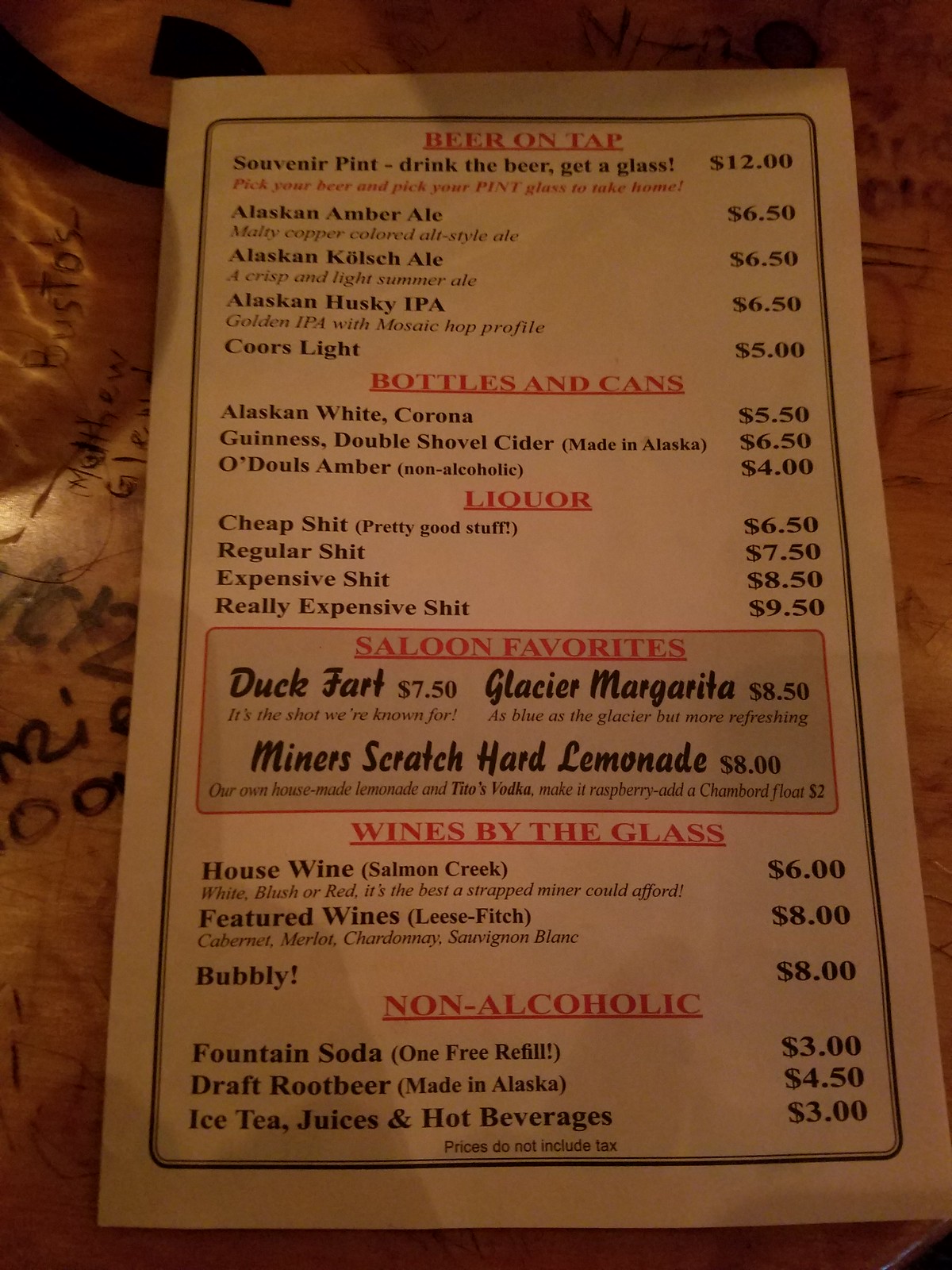This is a detailed photograph of a rustic drinks menu resting on a well-worn wooden tabletop. The menu features red headers and black text, categorizing the offerings into Beer on Tap, Bottles and Cans, Liquor, Saloon Favorites, Wines by the Glass, and Non-Alcoholic. The Saloon Favorites section highlights distinctively named drinks such as the Duck Fart, Glacier Margarita, Hard Lemonade, and Miner's Scratch. The Liquor section amusingly labels its selections as Cheap Shit, Regular Shit, Expensive Shit, and Really Expensive Shit, adding a touch of humor to the menu. The tabletop beneath the menu is heavily engraved and doodled with various markings, giving the scene a sense of history and character.